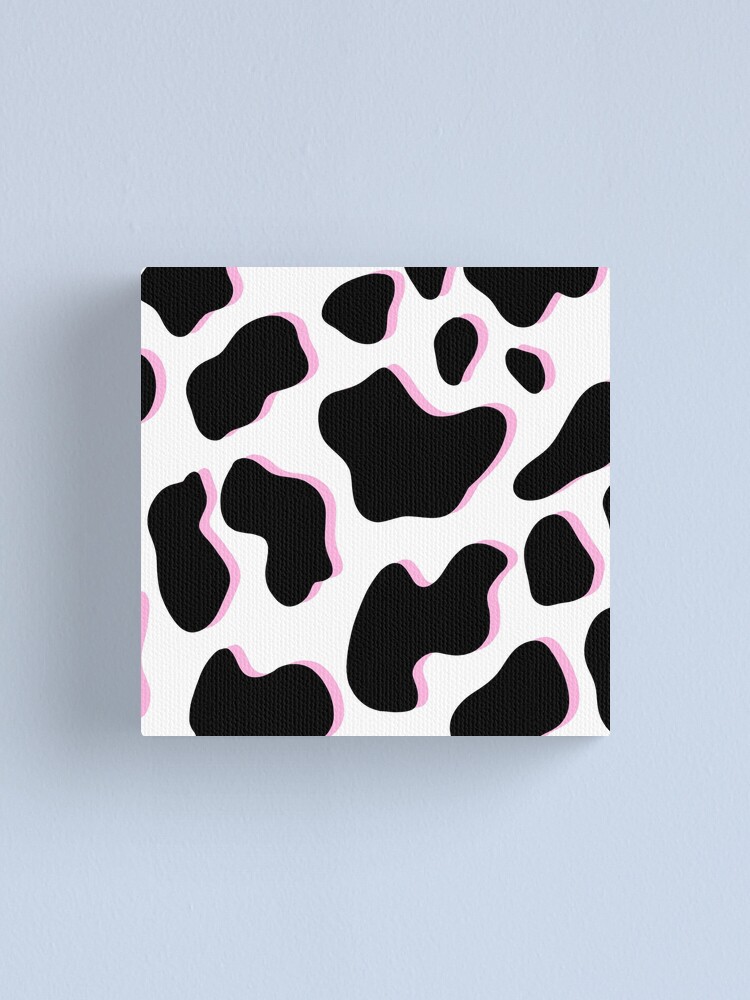The image depicts a square-shaped object, resembling a napkin or piece of art, situated centrally against a very light bluish-gray background. The square's background is predominantly white, adorned with random black spots that vary in shape and size, reminiscent of a cow's hide pattern. To enhance the three-dimensional effect, each black spot is outlined with pink shading, which gives an impression of depth and protrusion off the canvas. Soft, subtle shadows emanate from the black spots, mainly towards the bottom-left, adding to the dimensional appearance. This piece, evocative of contemporary art, lacks any textual elements, bringing focus purely to its visual patterns and spatial play.